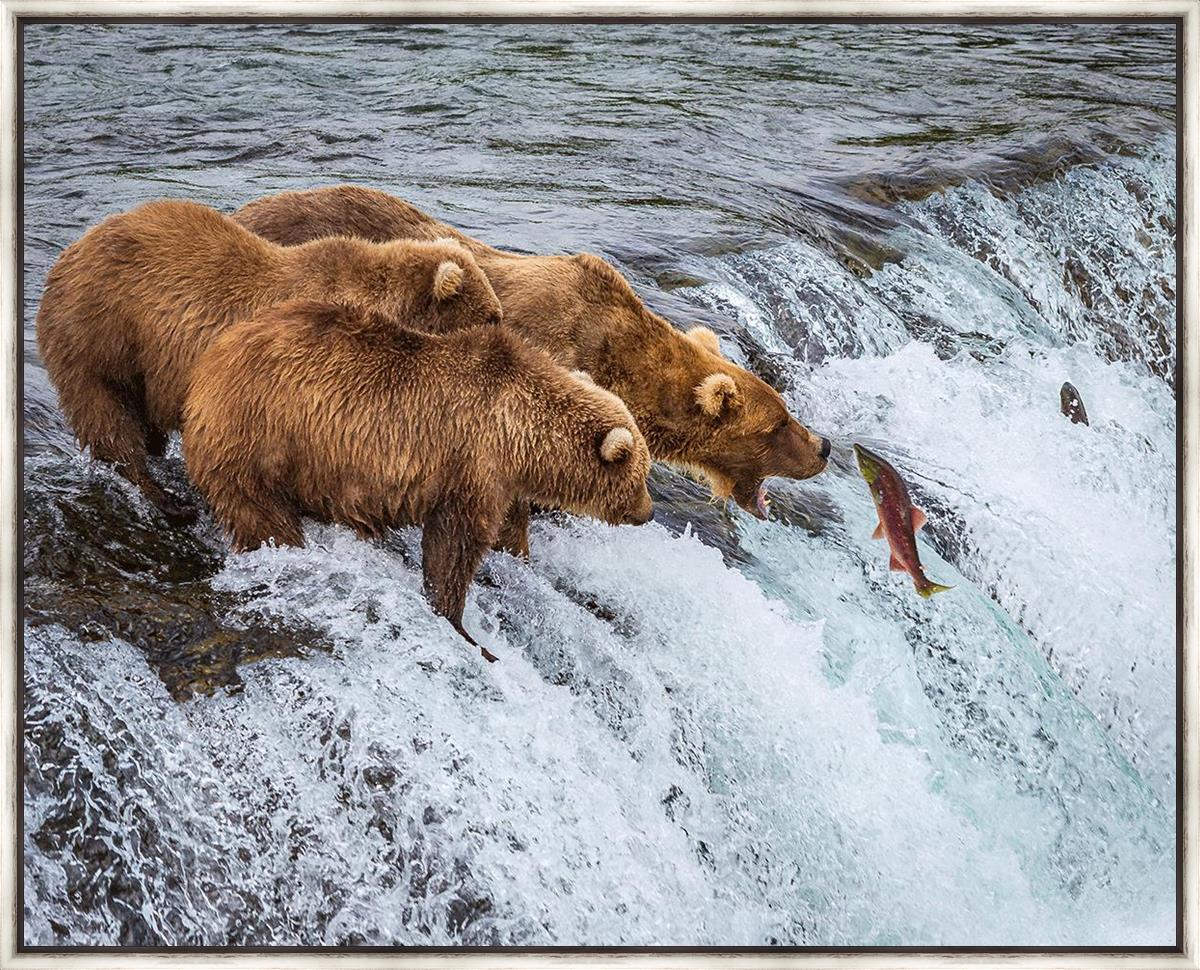This rectangular framed painting, measuring about 6 inches by 4 inches and bordered with a thin white and black frame, vividly depicts an outdoor scene featuring three brown bears at the edge of a small waterfall. The bears are centralized on the left side of the image, standing in a rocky area where the water cascades gently, transitioning into a frothy turmoil on the right. The bear closest to us stands facing right, while the second bear is slightly behind it. Another bear farther away is captured with its mouth wide open, poised to catch a fish leaping from the churning, white frothy water below. The fish, detailed with a green head and tail and a light reddish body, forms a focal point, suspended mid-air in this vibrant moment. The background of brown and green hues paints the serene top of the river behind the cascading waterfall.